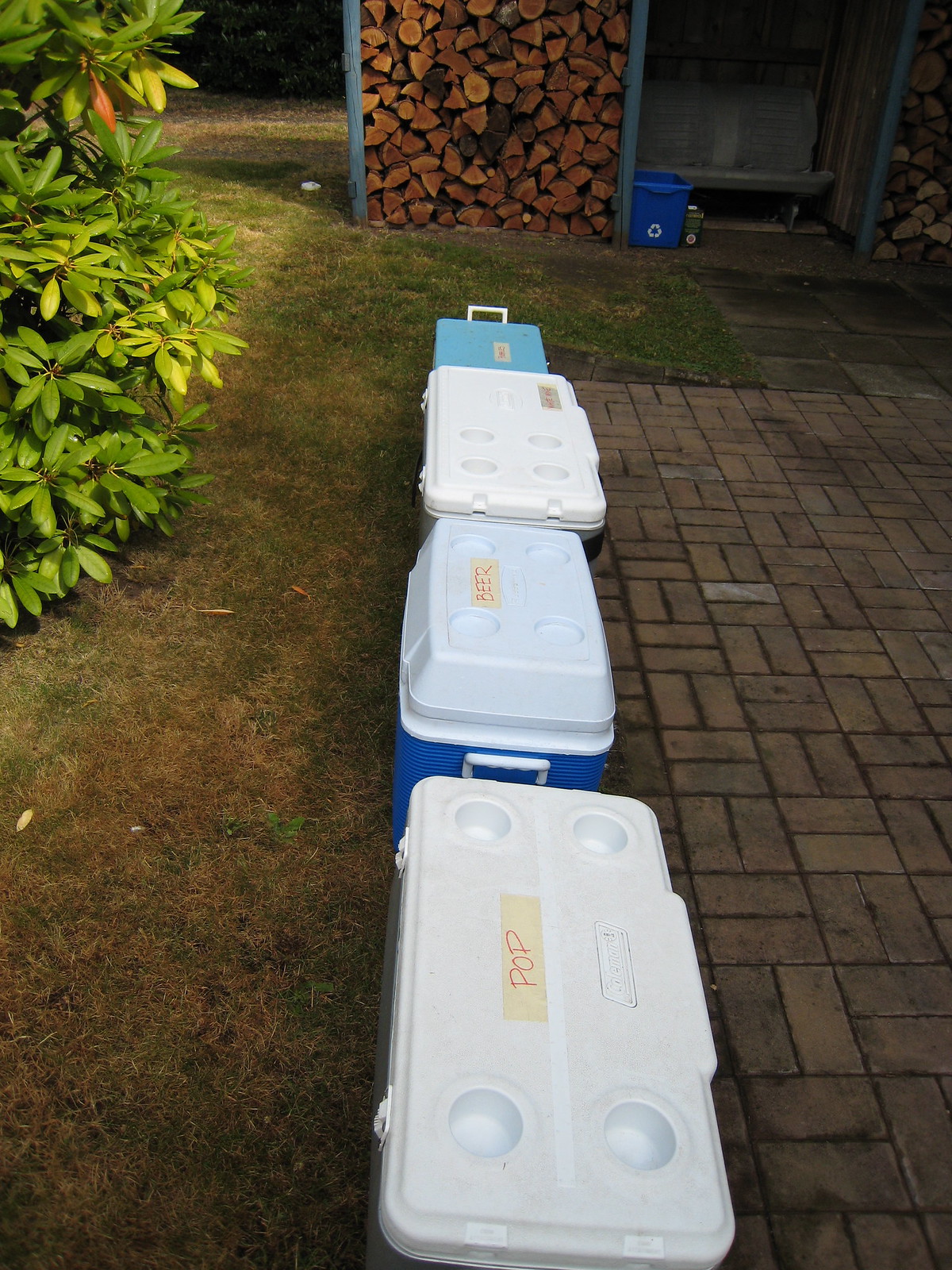The image captures a detailed scene set during what appears to be the late afternoon or evening, given the warm lighting. Central to the photograph is a brick patio where four sizable coolers are placed side-by-side. Each cooler has a white top and is labeled with tape; one reads "pop" and another "beer". These coolers are predominantly blue on the bottom. They are positioned near the edge of the patio, which itself is meticulously laid with rectangular bricks. To the back and one side of the patio resides a building constructed from logs of varying shades of brown, and some stored firewood is piled up, ready for use. In the middle right of the scene stands a large blue recycling bin marked with a white recycle symbol. Surrounding the patio is a patchy lawn of green grass interspersed with brown patches, indicating some dryness. Additionally, there is a lush bush with vibrant green leaves within the frame, contributing to the outdoor ambiance.